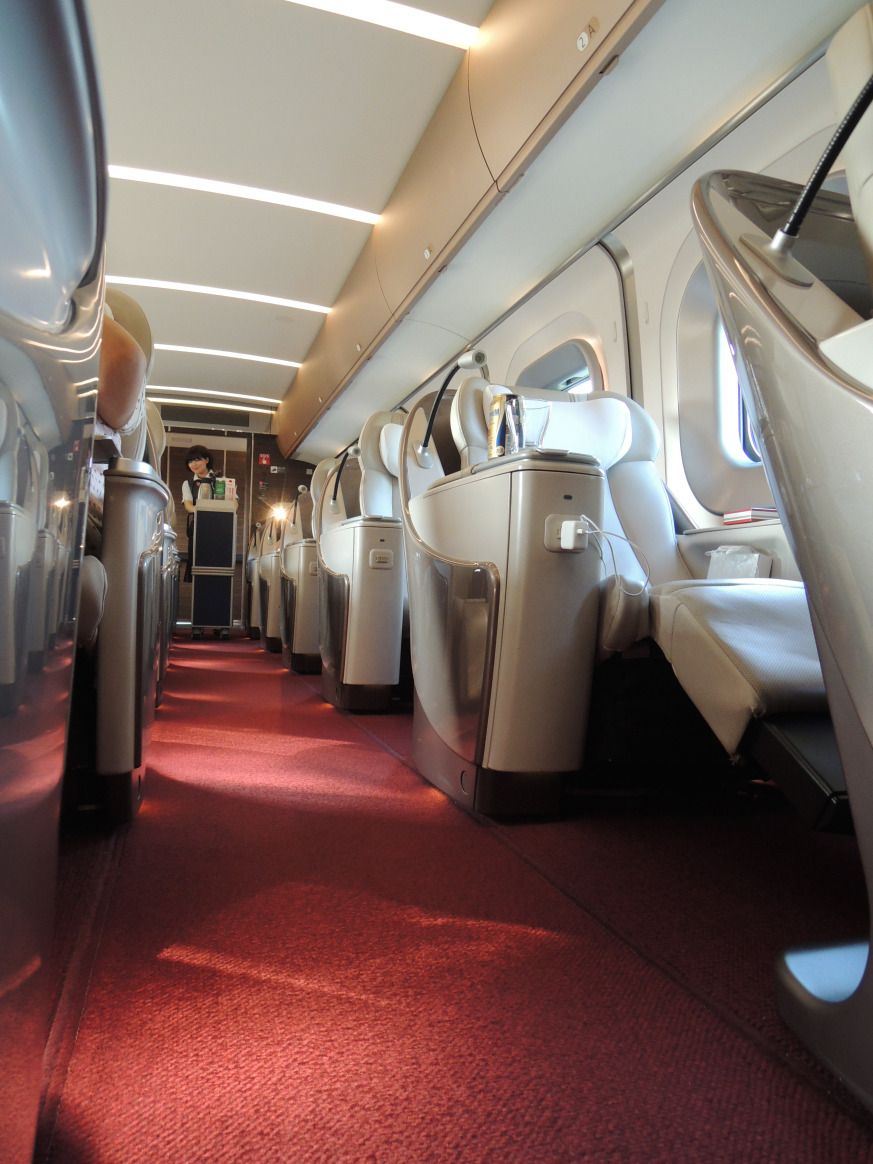The photograph captures the luxurious interior of a high-end, business-class airplane during the daytime, illuminated by a mix of natural and artificial light. The image is vertically rectangular and prominently features a red carpet running down the aisle. On both sides of the aisle are rows of off-white, cream-colored leather reclining seats, each seat standing alone without a partner. The right side of the image clearly shows airplane windows, an array of reclining seats, one of which has a footrest extended and a power brick plugged into an outlet beside it. A can of beverage, gold and blue in color, rests on the armrest of this reclined seat.

The seating area features maroon, orangey-red low-pile carpeting, adding to the opulent feel. Overhead, the ceiling is white, fitted with horizontal white light strips. The baggage compartments possess a bronzy tan finish with white sections underneath. At the back of the plane, a flight attendant with short dark hair and clad in a black and white uniform, likely of Asian descent, is seen pushing a drink cart. Another passenger is partially visible on the left-hand side, mostly obscured by a large, reflective metal object that dominates the left front part of the image, extending vertically.